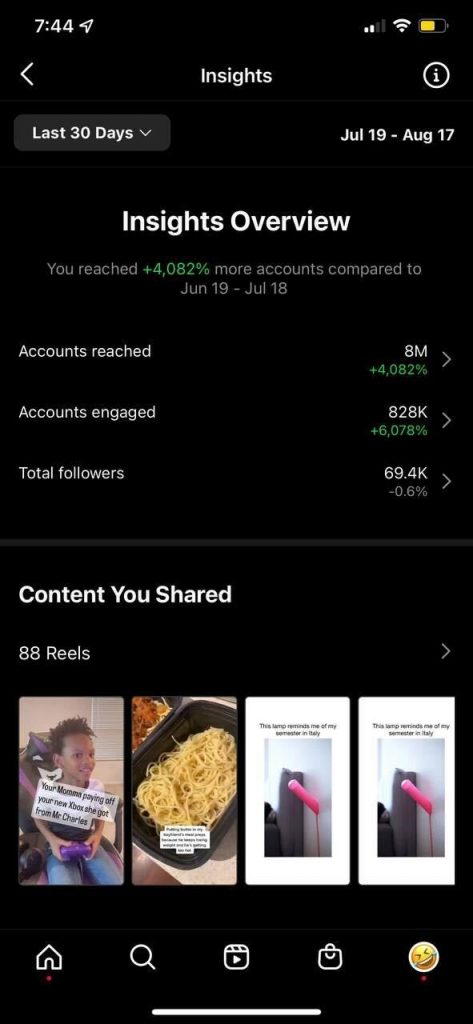This is a detailed screenshot of a cell phone displaying an "Insights Overview" screen. At the top of the screen, typical smartphone status indicators are visible, including a battery bar, signal strength bar, and a network speed indicator, confirming the device is a cell phone. Below these indicators, the user has navigated to the "Insights" section, as indicated by the title at the top and a back arrow for exiting this view.

The time frame for the insights is set to the last 30 days, specifically from July 19 to August 17. This "Insights Overview" provides metrics on the user's account performance such as the number of accounts reached, accounts engaged, and total followers. The data shows substantial interaction, indicating the user has a significant amount of engagement.

Further down, the screen displays content shared by the user, stating a total of 88 items shared, though only four thumbnail images are currently visible. These images provide a glimpse into the types of content shared and offer quick access for further insights on each item.